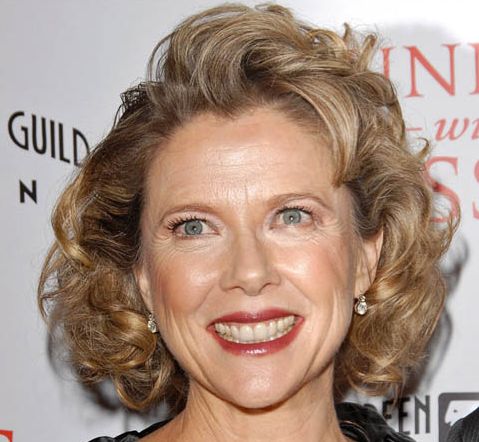The image is a neck-level photograph of Annette Bening, a strikingly beautiful woman with a classic Hollywood look. Her dark golden hair, styled in soft, coiffed curls with a right-side part, perfectly frames her face. She is adorned with makeup, including a light red lipstick accentuating her broad, open-mouthed smile that reveals her teeth, and her expressive gray eyes. Elegant white stoned earrings add to her glamorous appearance. Annette is dressed in what seems to be a dark, possibly black outfit visible at the bottom of her neck. She is standing in front of a white banner featuring partially visible black and red lettering, creating a subtle shadow behind her. The overall composition highlights her poised and timeless elegance against a textured backdrop.